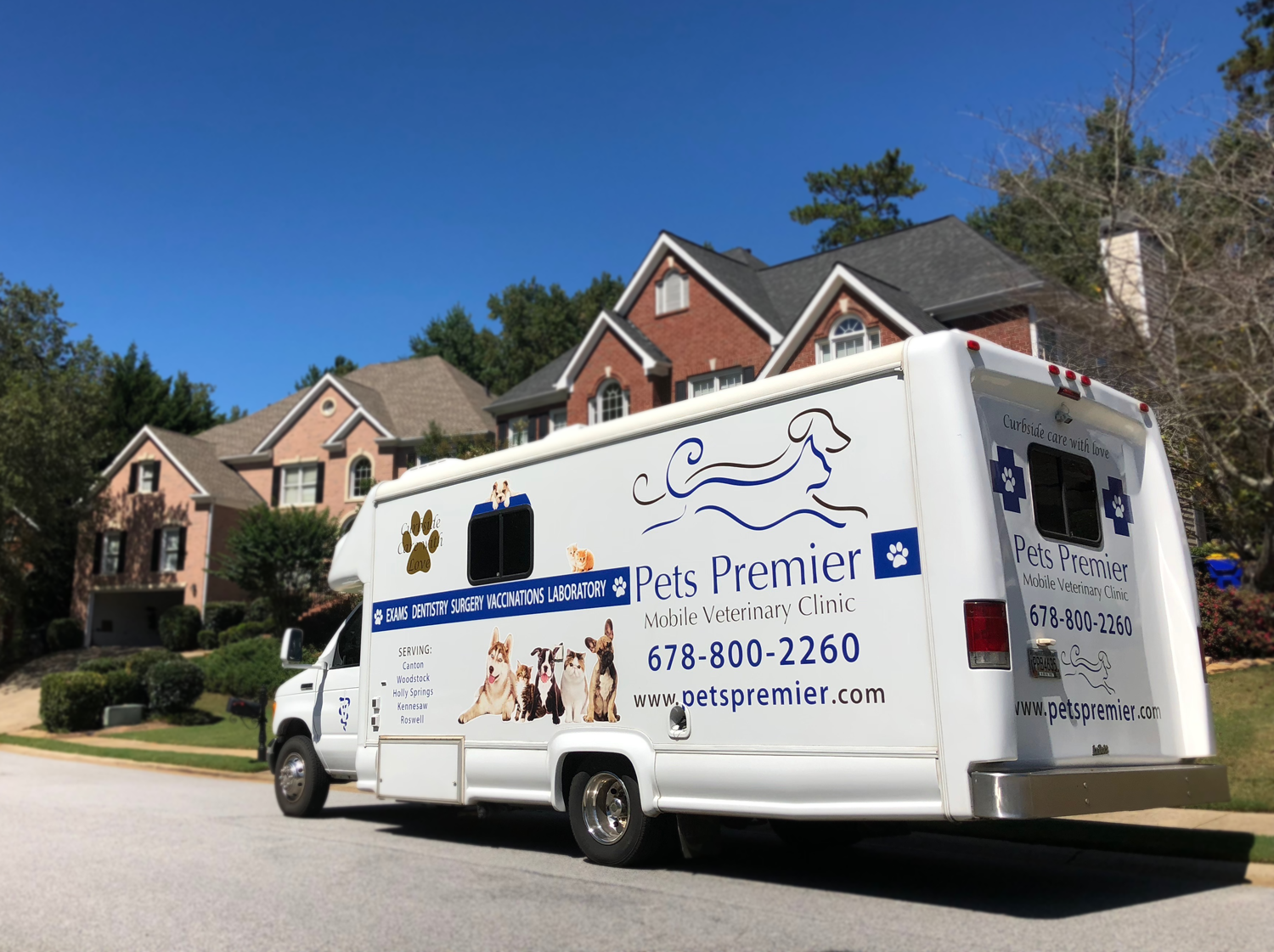In this brightly lit outdoor photograph, a large white van labeled "Pets Premier" is parked curbside in a suburban neighborhood. The van, which serves as a mobile veterinary clinic, displays various detailed graphics including a blue and black line art illustration of a running dog and cat, a blue square with a white paw print, and multiple images of different dog and cat breeds. Prominently featured on the side of the van are services it offers: exams, dentistry, surgery, vaccinations, and laboratory work. The contact details, 678-800-2260, and the website, www.petspremier.com, are clearly printed. The surrounding background reveals a clear blue sky, sunlight illuminating the scene, and two well-kept houses with landscaped gardens and smaller trees. One house has a dark brown brick exterior with white-framed windows and a grey roof, while the other features a light brown roof with mild pink walls. Both houses add to the picturesque suburban setting, enhancing the community-focused essence of the mobile clinic, which provides convenient curbside care for pets in cities like Canton, Woodstock, Holly Springs, and Roswell.